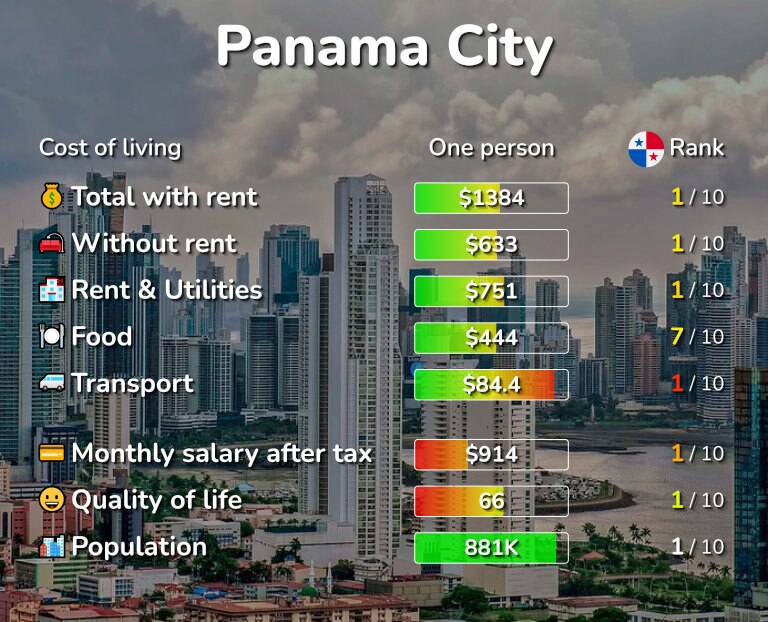The image titled "Panama City" portrays a skyline view of the city featuring prominent skyscrapers adjacent to a body of water, which could either be a river or the coastline of the ocean. The infographic displayed provides a comprehensive overview of the cost of living in Panama City, broken down into three columns: Cost of Living, One Person, and Rank.

The detailed breakdown is as follows:
- **Total Cost of Living for One Person (including rent):** $1,316
- **Cost of Living (excluding rent):** $607
- **Rent and Utilities:** $709
- **Food:** $426 (Ranked 3 out of 10 in terms of affordability; it's unclear if 1 is good or 10 is good)
- **Transport:** $78 (remarkably cheap)
- **Monthly Salary after Tax:** $901 (highlighting the stark reality that the average monthly salary is insufficient to cover rent)
- **Quality of Life Index:** 1 out of 67 (indicating poor quality of life)
- **Population:** Approximately 881,000

The image underscores the economic challenges faced by residents, where the cost of rent exceeds the average monthly salary, painting a grim picture of the living conditions in Panama City.